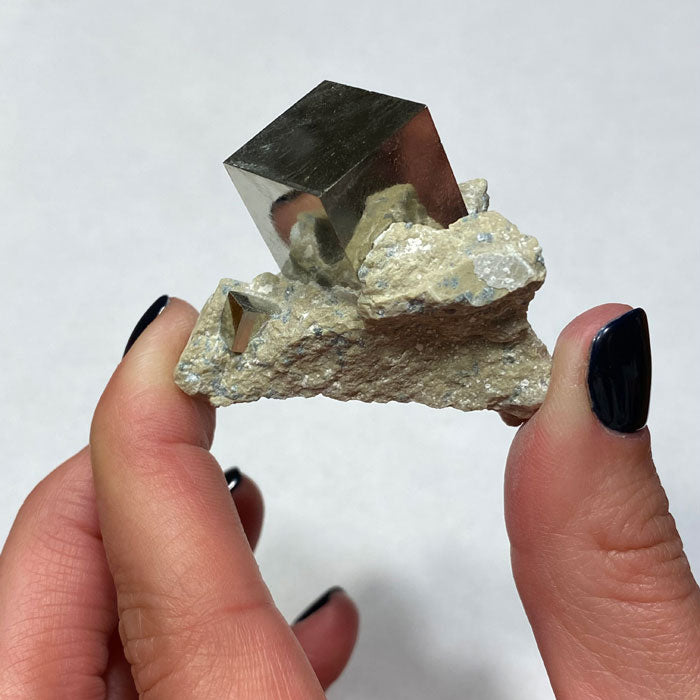The image depicts a left hand, with black-painted fingernails, holding a tan-colored rock embedded with a shiny, reflective mineral. The hand, which is missing its pinky finger, belongs to a person with light, pinkish pale skin. The rock is held between the thumb and index finger, appearing tightly gripped. The mineral embedded within the rock has a spherical shape and reflects the fingernails on the left bottom side. The background of the image is a plain gray or white, with the fingers casting a shadow in the bottom middle. There are also little patches of blue on the rock, and a distinctive black square-like design on the mineral, which enhances its reflective quality.